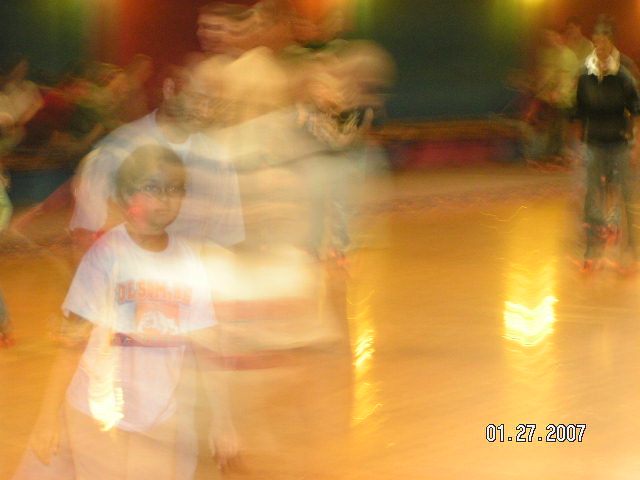The photo, taken on January 27, 2007, captures an indoor setting with orange-tiled flooring and a mix of green and red background elements. The image features various figures, all appearing blurred and ghostly due to motion blur. In the foreground, a young boy in glasses and a white shirt stands next to an older man, also in a white shirt. In the background, three people can be vaguely seen together, while another group sits in the top left corner. To the top right, a man in a black shirt with blue pants and a white collar appears to be pushing a stroller, accompanied by two others also pushing strollers. The date "1-27-2007" is faintly visible at the bottom of the image. Yellow lights are reflected on the floor, giving the scene a somewhat dreamlike quality.